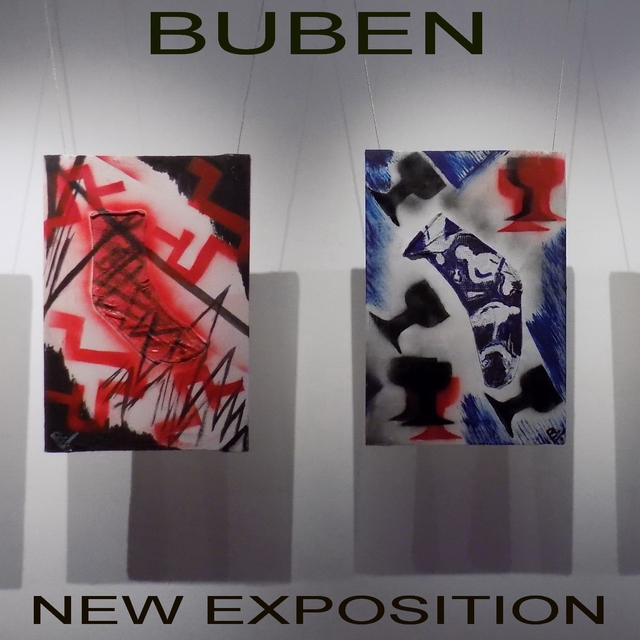This image features a striking art exhibition titled "BUBEN," displayed in bold, black, all-capital, sans serif font at the top of a pristine white wall. Below this title, the words "NEW EXPOSITION" are prominently displayed in the same font. Central to the exhibition are two evocative artworks, hung side-by-side by strings that cast shadows on the wall. The left painting, awash in a palette of red, black, and white, showcases a red sock adorned with black stripes at its center, surrounded by intricate decorations and flourishes. The right painting, primarily in blue, features a blue sock detailed with white silhouettes of people, and is encircled by small goblets in black and red. Both pieces incorporate a mix of freehand freestyle spray paint and stencil techniques, creating a dynamic and textured visual experience.